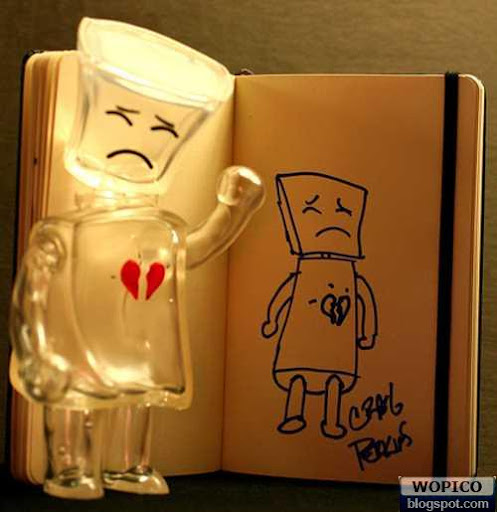The image depicts a clear glass figurine on the left side, set in front of an open notebook on the right. The figurine, resembling a small, human-like figure with a wide, square head, has its left arm raised in a fist. Its face shows closed eyes and a frowning mouth, conveying a sad expression. At the center of its chest is a prominent red heart, broken into two separated halves. The notebook features a line drawing of the figurine on its right page, mirroring the glass figure's sad face and broken heart but with both arms lowered. Additionally, the notebook is held together by a black ribbon on the right side, and the artwork is signed "Craig Paris" on the bottom right of the page.